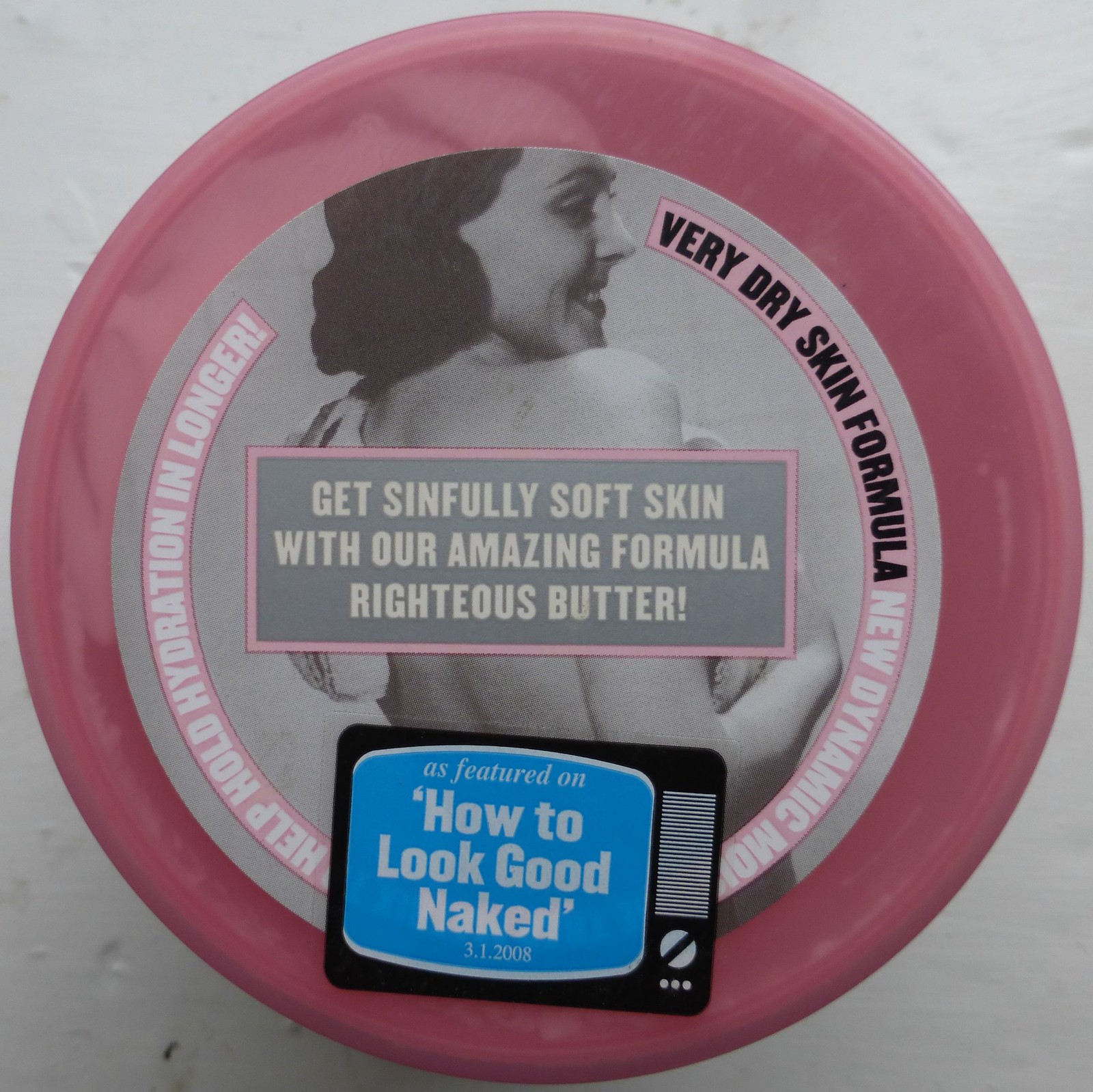The image captures the top view of a circular beauty product, likely a body butter, placed on a textured white surface. The product itself is a pleasing bubblegum pink color with a central round sticker. The sticker features a retro, black-and-white image of a woman from the 60s, smiling and looking to the right. She appears to be draped in a towel, with some portions of her image obscured by other design elements. Surrounding her image are various pieces of text: "Very Dry Skin Formula," "New Dynamic," “Get Sinfully Soft Skin with our amazing formula Righteous Butter,” and "Help Hold Hydration in Longer." An illustration of an old television is also present on the sticker, with text on the screen reading "As featured on How to Look Good Naked, 3-1-2008.”